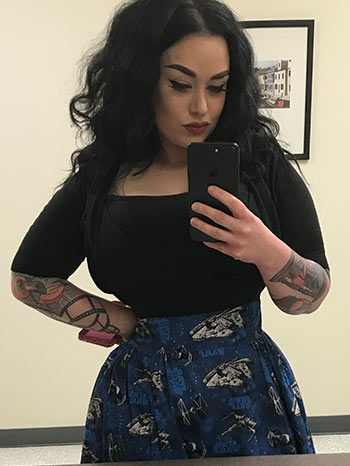In this realistic, vertically oriented photograph, a woman with light skin and wavy black hair stands inside a room with light beige walls adorned with a black-framed city landscape picture with a white matting. The wall has a dark trim, and the floor is light beige. The woman appears to be in her 20s or 30s, wearing black eyeliner, black eyebrows, and red lipstick. She is dressed in a black top with elbow-length sleeves and a square neckline, paired with a predominantly navy blue skirt featuring white and dark blue patches. Her arms are adorned with tattoos in colors like black, red, and light gray, with one on her left arm resembling a wrap and something pink hanging off her right wrist. She is holding a black cell phone in her left hand, looking at it as if she might be taking a selfie, and a phone case cupped in her right hand at waist level. The picture behind her and her detailed appearance create an intriguing, candid moment centered around her interaction with her phone.